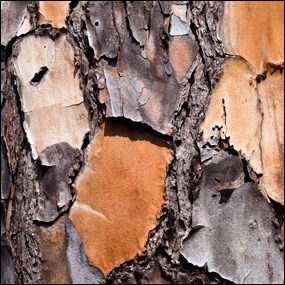The image is a detailed, tightly framed, color photograph of a tree trunk showcasing the intricate textures and colors of its bark. The bark exhibits an array of hues, ranging from varying shades of brown, dark brown, and rust-like orange to lighter tones of tan, cream, and gray. It features several distinct sections: a central portion where the bark has peeled away, revealing darker wood beneath; an orange segment on the right side with additional peeling; and an area of predominantly white bark also on the right. A vertical element in dark gray runs from the top, resembling a shingle, while an orange, oval shape emerges from the bottom. The upper right displays light orange tones layered over gray, and there is a beige form on the top left. Some bark curls up at the bottom right, mimicking burnt gray paper. The image captures these textures and colors with photographic realism, filling a small square frame entirely with the rugged beauty of the tree's surface.